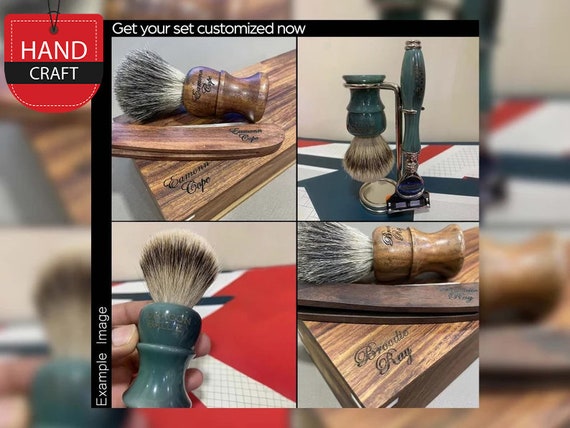This image appears to be a detailed promotional advertisement for a custom-made shaving kit, possibly found online or in a magazine. The advertisement features two overlapping photos. The larger, background image is somewhat fuzzy, while the smaller, front image showcases the shaving kit in various close-ups. The header of the front image has a black border with the text "Get Your Set Customized Now." 

A tag on the upper left-hand corner reads "Handcraft" in white text on a red background, accentuated by a black stripe. Below this tag is an example image showing a wooden box with an engraved name and an old-fashioned shaving brush featuring fine, soft bristles. The brush handle appears wooden, but other versions, including one blue non-wooden handle, are also shown. These brushes sit against a red and white patterned cloth. 

On the right side of the smaller image, multiple shaving brushes arranged in a stand evoke a vintage aesthetic. The bottom right corner of the image displays another variant of the shaving brush on a wooden box, though the text on the box is not legible. 

Additionally, the set includes both traditional shaving implements, such as a straight razor, and more modern options like a safety razor. This advertisement emphasizes the customizability and handcrafted quality of the shaving kit, making it an attractive option for those seeking a personalized and elegant grooming experience.